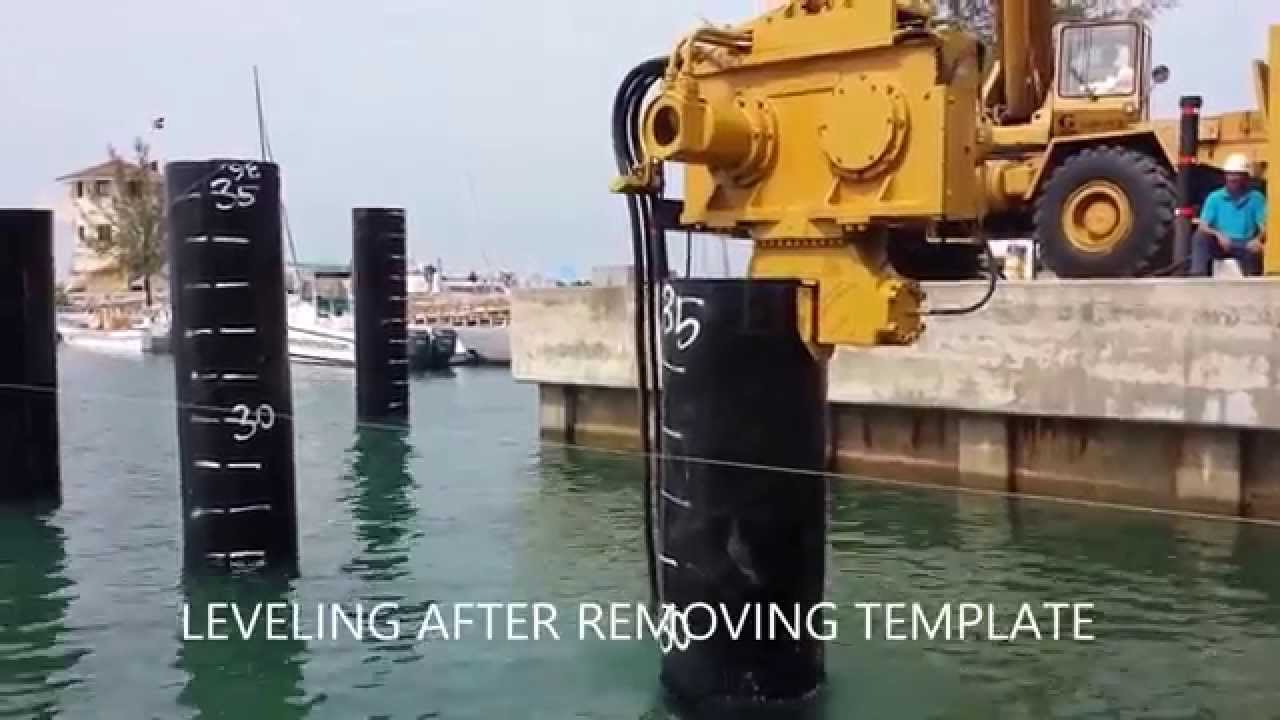The photograph captures a bustling dock scene where a large yellow truck is stationed on a concrete platform adjacent to a blue-green waterway. The truck appears to be attached to a substantial yellow pumping apparatus engaged in an unspecified pumping operation. Prominently, the dock features tall black pylons protruding from the water, marked with numerical depth indicators, presumably in feet, which measure up to 35 feet. The scene includes a man in a turquoise polo shirt and white hard hat overseeing the activity, seated on the dock. In the background, a variety of boats, including both sailboats and motorboats, are anchored near a boathouse, lending a nautical ambiance to the setting. The sky above is a light, featureless gray, contributing to the overall industrial yet serene atmosphere by the water.